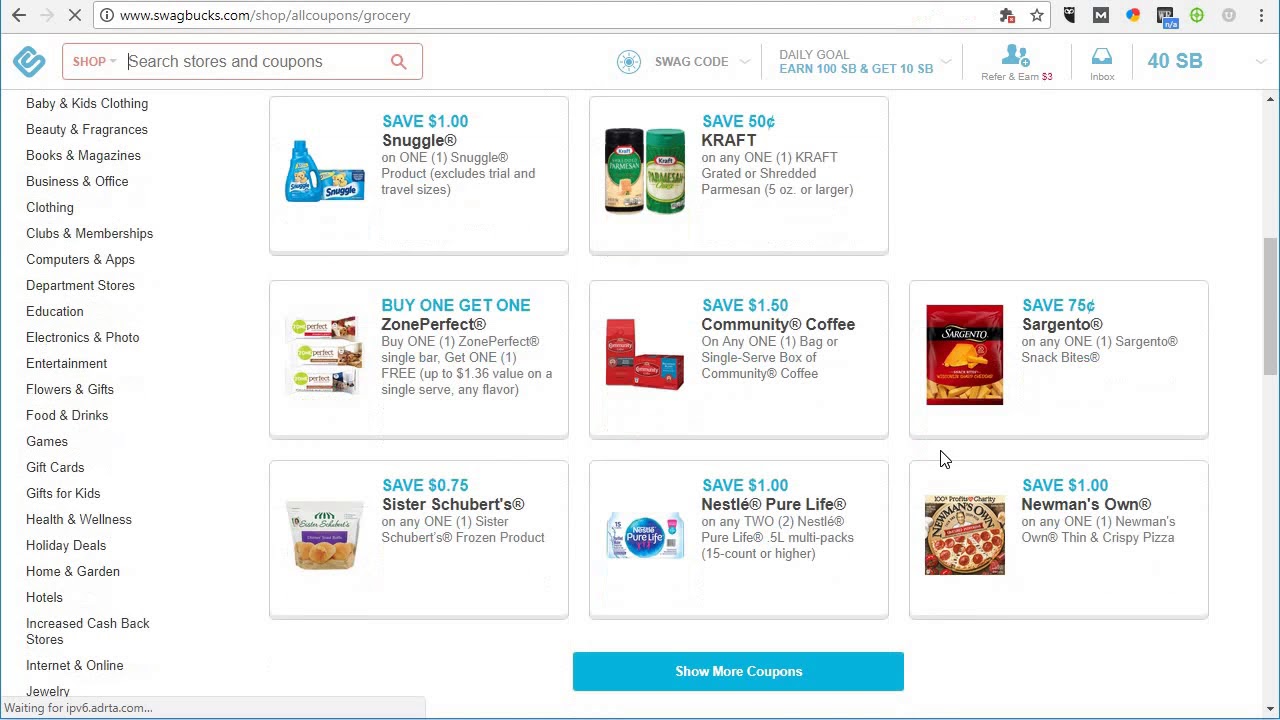The image depicts the Swagbucks website, focusing on the section featuring grocery coupons. At the top of the page, the URL reads "www.swagbucks.com/shop/all-coupons/grocery". The user currently has 40 Swagbucks, prominently displayed in blue. Additional navigation options include "Inbox," "Refer & Earn," "Daily Goal," and "Earn 100 Swagbucks and get 10 Swagbucks." There is also an input field for Swagcodes.

On the left-hand side, the menu displays options such as "Shop," "Search Store," and "Coupons." The search bar is highlighted with a red "Shop" label and a red magnifying glass icon. The Swagbucks logo is positioned on the left.

The central part of the page showcases various coupons with clickable images. Examples include:

1. **Snuggle Fabric Softener:** - "Save $1 on one Snuggle product (excludes trial size)." Image depicts Snuggle fabric softener.
2. **ZonePerfect Bars:** - "Buy one ZonePerfect single bar, get one free." Image shows a ZonePerfect bar.
3. **Sister Schubert's Frozen Products:** - "Save $0.75 on any one Sister Schubert's frozen product." Image depicts the product.
4. **Kraft Parmesan Cheese:** - "Save $0.50 on any one Kraft grated or shredded Parmesan cheese." Image shows Kraft cheese.
5. **Community Coffee:** - "Save $1.50 on any one bag or single serve box of Community Coffee." Image depicts a bag of Community Coffee.
6. **Nestle Pure Life Water:** - "Save $1 on any two Nestle Pure Life 5-liter multipacks, 15 count or higher." Image shows the water bottle.
7. **Sargento Snack Bites:** - "Save $0.75 on any one Sargento snack bite." Image depicts Sargento cheese.
8. **Newman's Own Pizza:** - "Save $1 on any one Newman's Own thin and crispy pizza." Image shows the pizza.

At the bottom, a blue icon reads "Show More Coupons," and a gray scroll bar is observable to the right.